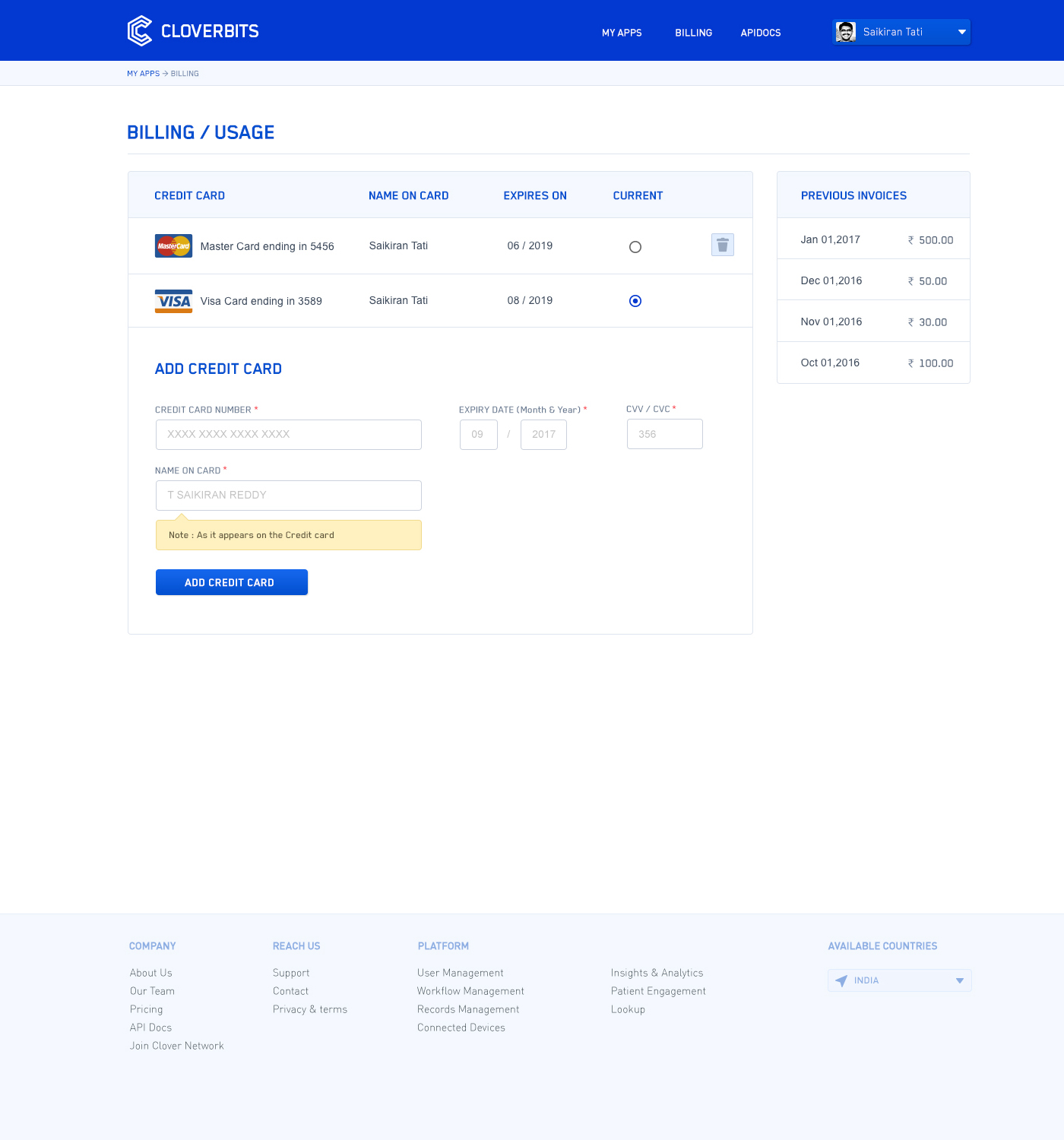This image is a screenshot from the Clover Bits website. In the top left corner, there is a blue navigation bar featuring the Clover Bits logo—a stylized white "C"—followed by the site name "Clover Bits." On the top right of the bar, there are navigational options, including "My Apps," "Billing," and "API Docs," adjacent to the user's information. The user's profile displays a picture of a man, likely of Indian descent with black hair and a mustache, named Sakirantati. A dropdown menu next to his name allows for profile-related actions.

Below the navigation bar, there is a secondary menu indicating that "My Apps" is highlighted in blue while a light gray arrow points to "Billing," suggesting the current section. The main content area begins with the title "Billing / Usage" in blue font, bordered by a light gray line beneath it. 

Further down, the billing information is organized into several boxes. The top left box is labeled "Credit Card," displaying fields such as the card type, name on the card, and expiration date. The first card listed is a MasterCard ending in 5456 under the name Sakirantati, expiring in June 2019; it is marked as not current, indicated by an unchecked circle and accompanied by a trash can icon for removal. Below that, a Visa card ending in 3589, also under the name Sakirantati and expiring either in June or August 2019, is shown as the current payment method, without a trash can icon for deletion.

At the bottom of this section, there's an option to add a new credit card. To the right of the credit card information, there is a list of previous invoices, dated January 1, 2017, December 1, 2016, November 1, 2016, and October 1, 2016.